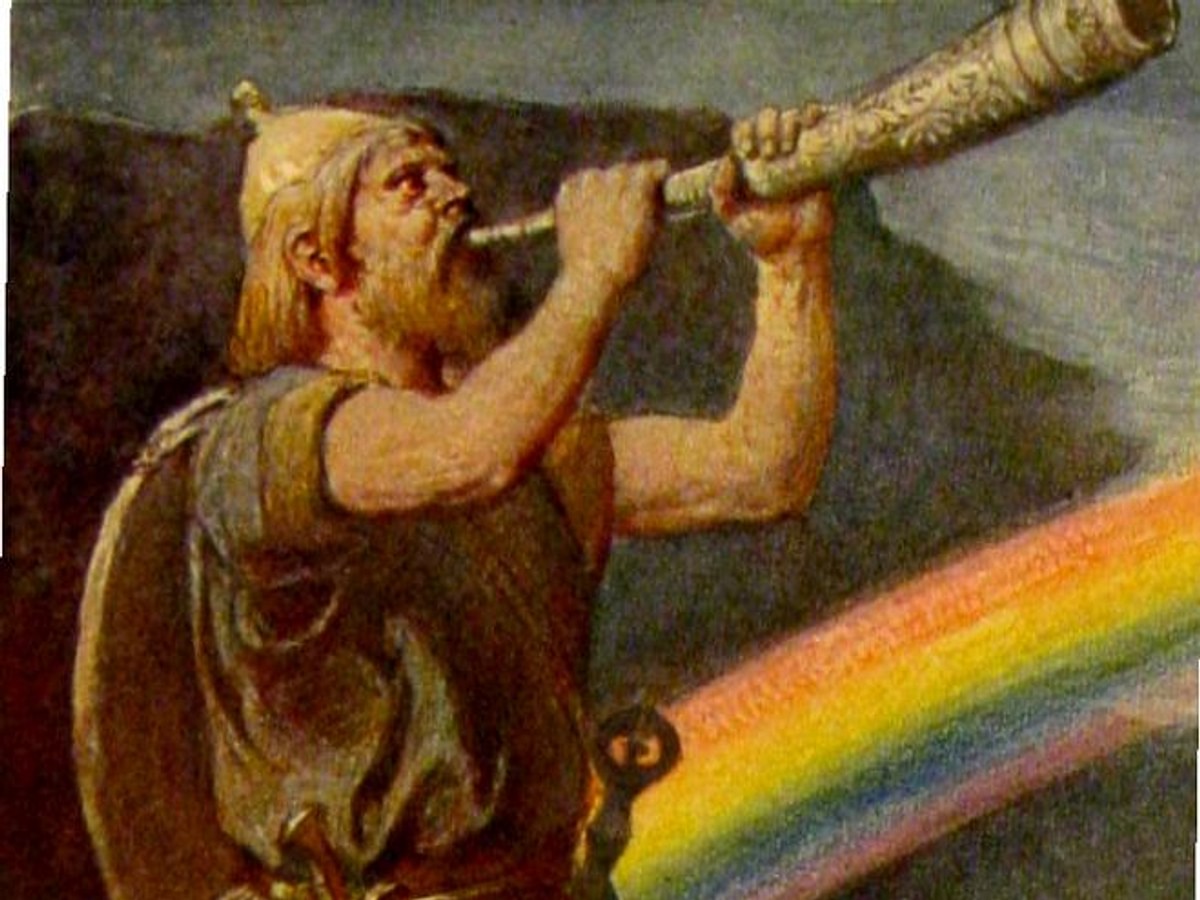In the artwork depicted, there is a somewhat blurry, yet captivating image that appears to be either a painting or a detailed pencil or pastel drawing. The focus of the artwork is a Viking figure adorned in a gray or possibly dark blue tunic. This Viking is portrayed with a shield strapped to his back and is wearing a small, pointed metal helmet. His long, flowing blonde hair and equally long, blonde beard add to the authenticity of the character. 

He is seen blowing an ornate horn, which is drawn or painted to give the impression of being made from metal and is elaborately decorated with intricate designs. The artwork also features a vibrant rainbow emerging from behind the Viking, adding a mystical and magical element to the scene. There is no text present in the image, allowing the striking visual elements to stand out prominently.